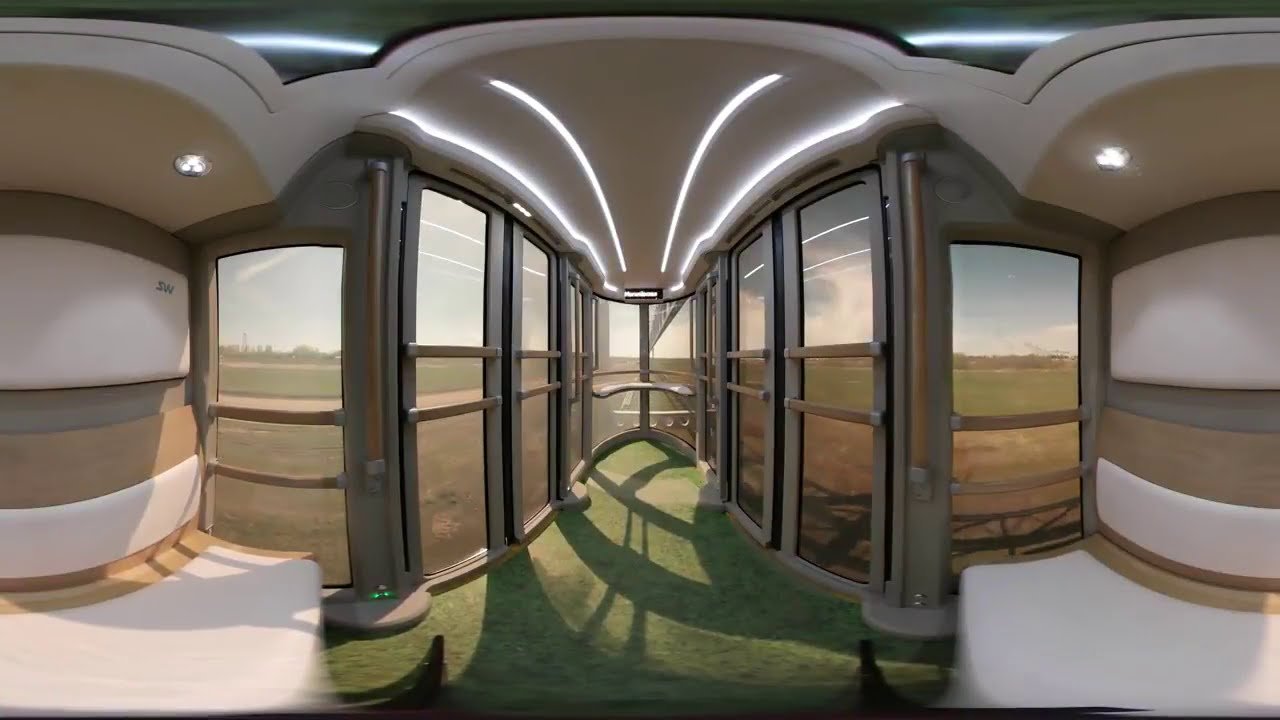The image depicts a futuristic, modern living space, seemingly a computer-generated portrayal of an interior. At the heart of the scene is a short, carpeted hallway adorned with green carpet, leading the observer's eye towards a central viewing area dominated by expansive windows. The windows provide glimpses of a serene countryside with blue skies, grassy fields, and tan patches of dirt.

Flanking the hallway, on the left and right, are built-in white and tan leather couches that curve elegantly along the walls. The walls themselves are gray, and the ceiling is domed and futuristic, embedded with slender, elongated lights that enhance the space's modern aesthetic. This central viewing area, designed as an observatory nook, features two prominently curved windows at the end, offering a panoramic vista.

The combination of green carpeting, white and tan seating, and the abundance of natural light streaming through the windows, coupled with the sleek, sci-fi architectural details, exudes a blend of sophistication and tranquility, capturing the essence of a luxurious, contemporary living space.